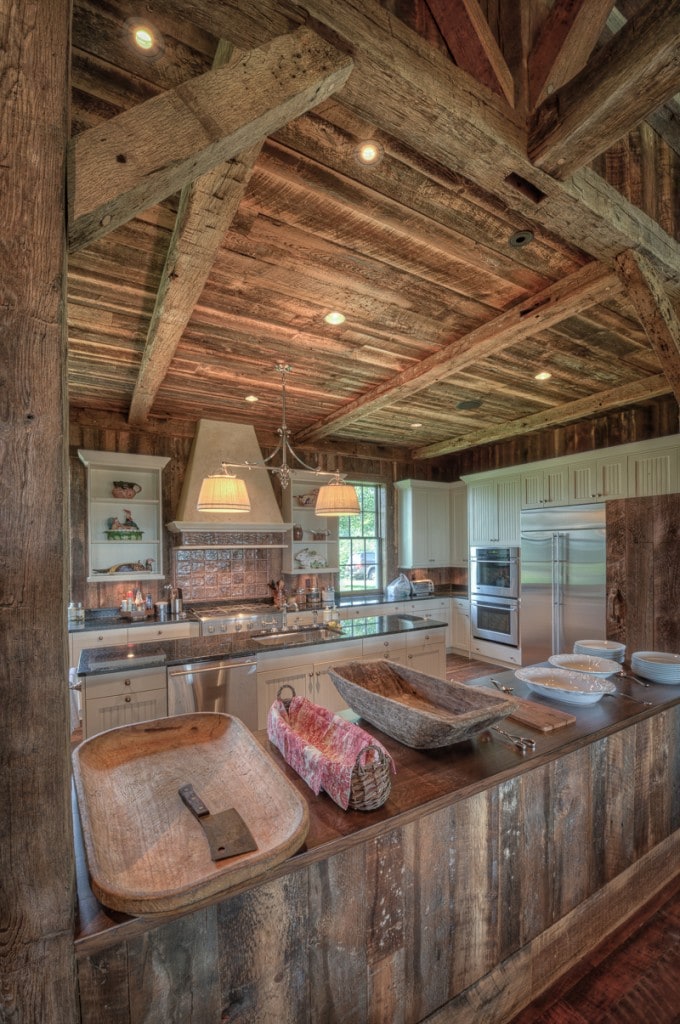The image depicts a bright and clear kitchen with a distinct woodsy atmosphere. The space features wooden elements prominently, including a wood plank ceiling with recessed lighting and a wood countertop. The kitchen is equipped with white-painted cabinets beneath the countertop, a stainless steel refrigerator, oven, dishwasher, and a kitchen sink with a white faucet and stainless steel fixtures. On the wooden countertop, there's a variety of food preparation items laid out, possibly indicating a large meal in preparation. These items include large dish bowls covered in plastic wrap, stacks of plates, a cutting board with a knife, and a wooden tray and basket. The kitchen walls appear to be wood-paneled, enhancing the rustic aesthetic. No people are visible in the image.